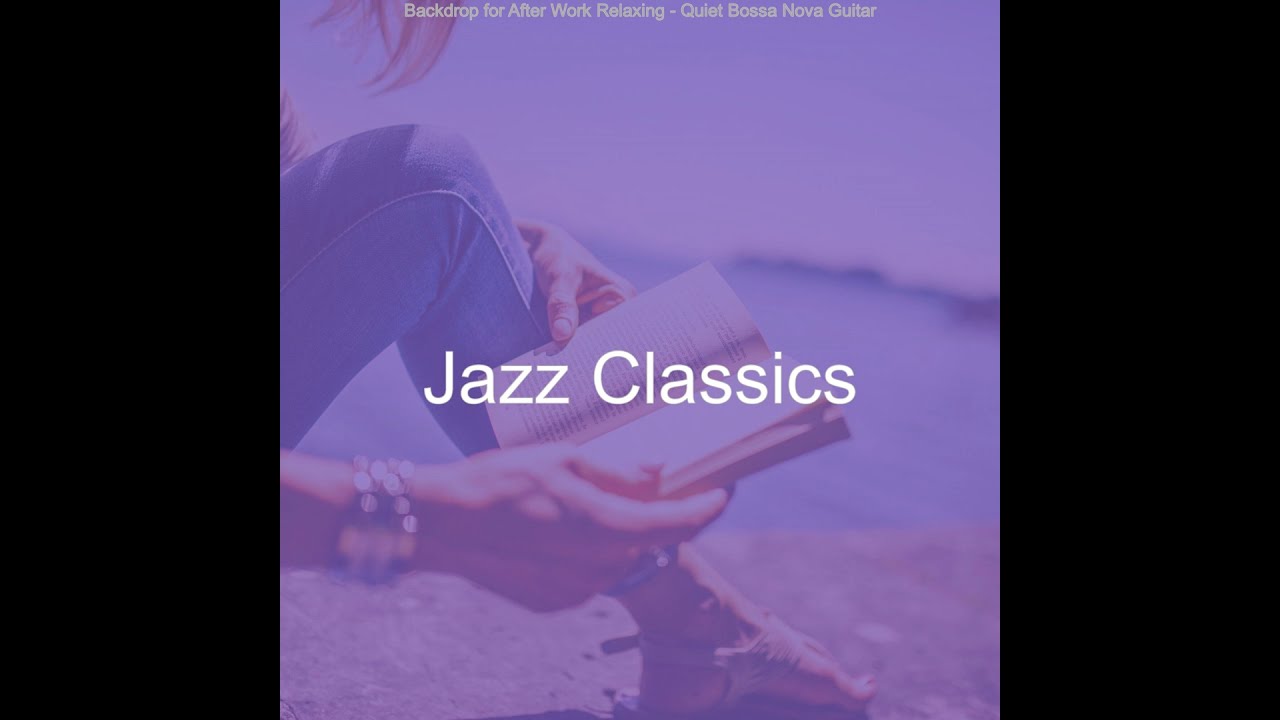In this image, we see a woman seated on what appears to be a sandy beach, with a serene backdrop suggesting a lake or ocean in the distance. The overall scene is filtered in a purplish hue, adding a tranquil, dreamy quality to the picture. The woman is dressed in blue jeans and sandals, with one leg bent at the knee, her foot pointing towards the bottom right of the image. Her left hand is wrapped around her leg, resting on the upper calf, while her right hand, adorned with a bracelet, holds the other side of an open book positioned at the center of the frame. A few locks of her hair are visible at the top left of the image. The text overlays the scene in white letters, with the phrase "Jazz Classics" prominently centered. Above that, in smaller print, it reads, "Backdrop for After Work Relaxing, Quiet Bossa Nova Guitar," emphasizing the mellow, soothing atmosphere perfectly suited for unwinding after a long day.